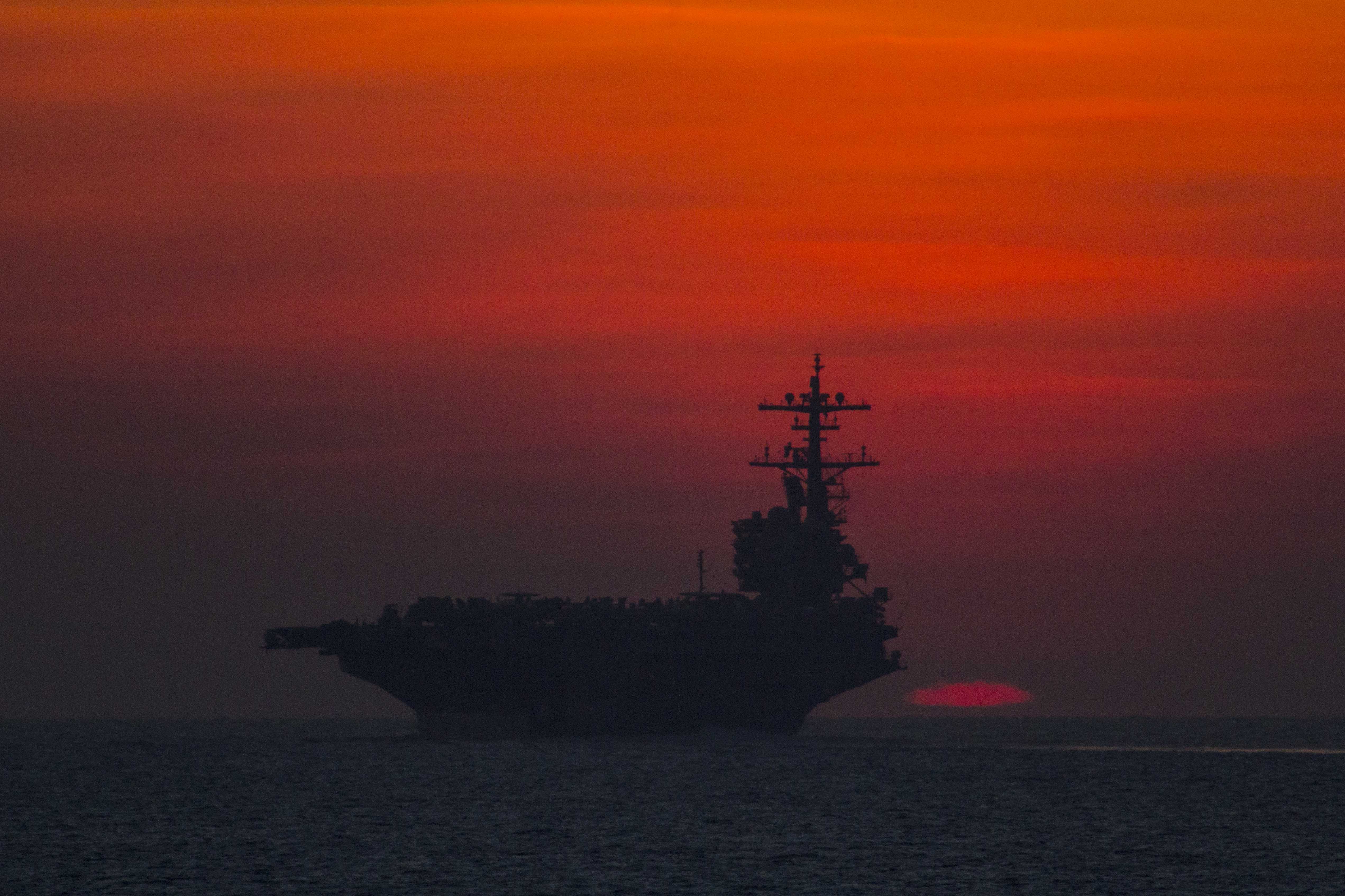The photograph captures a large battleship at sea, taken during either sunrise or sunset, with the very top of the sun peeking over the horizon to the right of the ship. The sky displays a brilliant gradient from dark, fiery reds and bright pinks near the horizon, transitioning to a darker purple hue as it ascends. The silhouette of the ship dominates the scene, outlined starkly against the vibrant center of the sky, emphasizing its imposing size and structure. The battleship, almost pitch black due to the lighting, faces left with a tall mast at the back, possibly equipped with antennas or various equipment, and a sizable, building-like structure on top. The deck appears jagged and rugged with indistinct piles, maybe crab pots or other stacks, adding to its intricate silhouette. The calm sea, devoid of land, features only small, gentle waves, enhancing the stillness and solemnity of the moment. The entire composition draws the eye to the striking interplay between the dark ship and the colorful, luminous sky.